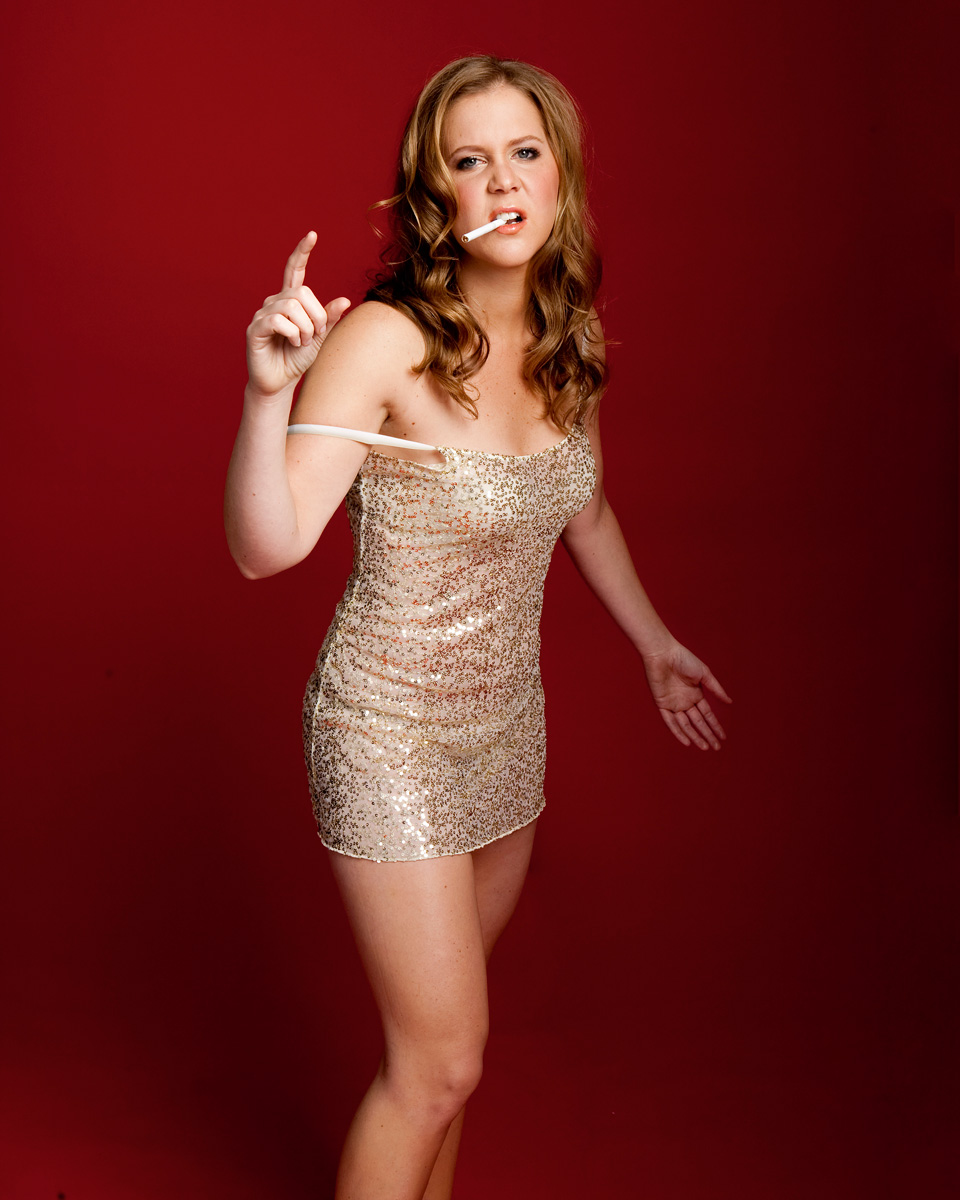In this striking photograph, actress and comedian Amy Schumer is captured from the mid-calf upwards, centered against a red background that transitions to darker shades, almost black, around the edges. She faces the lower right corner, yet her gaze fixates directly at the camera with a slight scowl of attitude. Schumer’s long, curly blonde hair flows past her shoulders, parted near the center.

She sports a provocative, thin-strapped, cream-colored sequin dress with one strap suggestively slipped off her shoulder. The dress glimmers with gold accents, hugging her frame tightly and ending just below the point where the crop cuts off the image. Her right arm is bent at the elbow, pointing upwards with her index finger extended while her other fingers are curled inward. Her left hand rests open-palmed by her side. A white, unlit cigarette dangles from her lips, accentuating her fierce, rebellious demeanor against the solid, shadowed red backdrop.